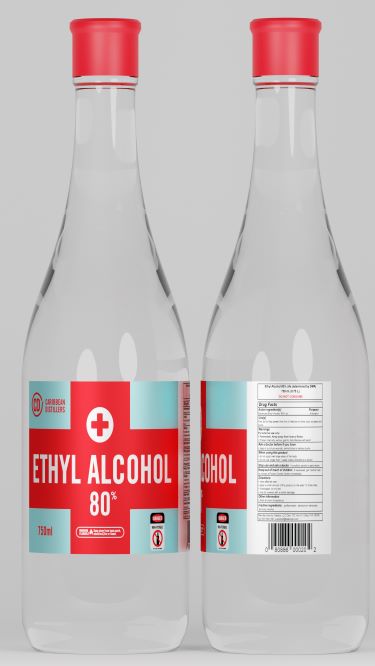The photograph depicts two tall, skinny, transparent glass bottles of ethyl alcohol, each capped with a red lid, standing upright against a gray background. The bottle on the left fully faces forward, showcasing its detailed label, which features a prominent red cross within a white circle set against a teal background. The text on this label reads "Ethyl alcohol, 80%" in white lettering, with a smaller, somewhat obscure warning label and a red "750 ml" indication on the lower left. The brand name is positioned on the upper left, though it is difficult to discern. The bottle on the right is angled slightly, revealing a white warning sign and possibly ingredient information. Both bottles suggest a medical context and remain unopened. The image's color palette includes gray, red, teal, white, and black.